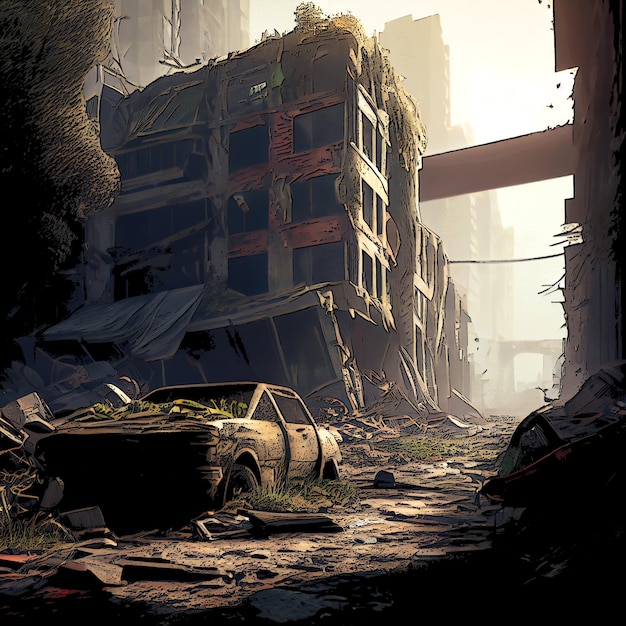This digitally rendered image depicts a post-apocalyptic cityscape reminiscent of visuals from video games or comic books, drawing parallels to scenes from movies like "I Am Legend" or "Mad Max." The bottom third of the image features a cracked, concrete street interspersed with patches of growing grass. On the bottom left, there's a derelict car, devoid of windows and partially reclaimed by nature with plants growing inside and around it. Central to the composition, slightly to the left, stands a dilapidated building with broken windows and vegetation creeping up its facade. In the distant background, two skyscrapers loom—one centered toward the top and another in the top left corner—adding depth to the scene. The leftmost part of the image, in front of the old building, showcases a lone tree. The overall color palette is a mix of gray, brown, green, black, yellow, and white, with flashes of red highlighting some building structures. The image captures a desolate, destroyed urban environment where nature is gradually reclaiming the ruins, with scattered debris and exposed infrastructure like hanging wires and rebar, suggesting a world where civilization has collapsed and the remnants are slowly being overtaken by the encroaching greenery.